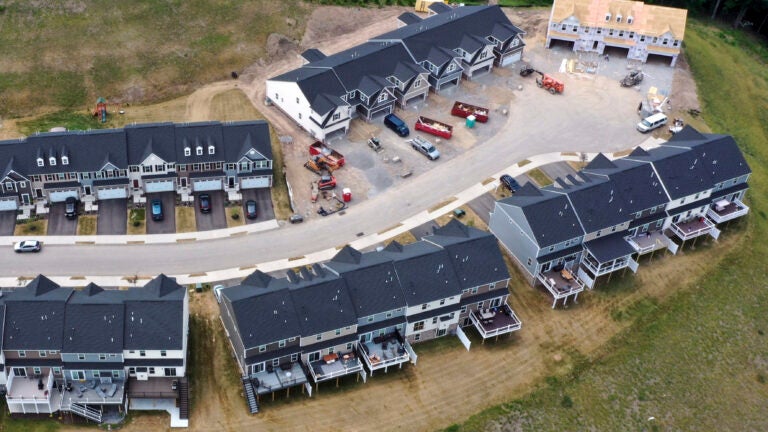The image captures an aerial view of a newly developed residential neighborhood set amid a vast, bare field, isolated from visible civilization. It showcases a cul-de-sac at the center, with multiple sets of townhomes and standalone houses, all featuring navy blue and charcoal gray roofs, except for a beige house with white trim in the middle of the cul-de-sac. Most homes appear occupied, evidenced by cars parked in their driveways and items like grills and chairs on the decks. Some areas, particularly around two units, are under construction; one unit is nearly complete while the other is far from finished. Construction equipment, dumpsters, and cranes are visible around these incomplete structures. The yards are still developing, with some patches of grass. A sidewalk runs along the right side of the main paved road, and a vehicle is seen driving down the street on the far left. Overall, the image captures a blend of newly inhabited homes and active construction amidst a large, open field.